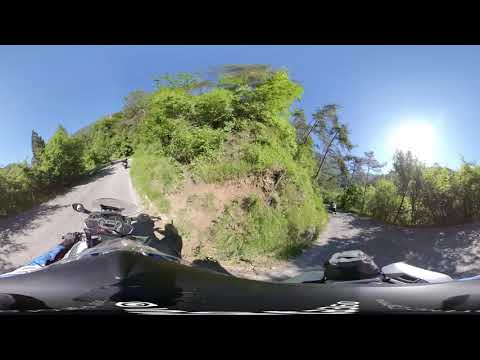This outdoor photograph, taken with a fish-eye lens from the perspective of a helmet camera on a motorcycle, captures a vivid scene on a winding country road. The black motorcycle is positioned on the left of the image, with the rider's blue-gloved hand visible. The asphalt road, tinged with gray, curves left around a small hill adorned with lush greenery. Bushes and trees, displaying varying shades of light and dark green, are scattered across the hill's landscape. In the distance, a black or gray vehicle is faintly visible ahead on the road. To the right, additional road curves around the hill, leading the viewer's eye toward the horizon. The sky is a clear, bright blue, with the sun positioned on the right, casting long shadows that suggest the time is either early morning or late afternoon. The overall effect of the fish-eye perspective gives the scene a slightly distorted but dynamic view, emphasizing the open, natural setting and the rider's vantage point.